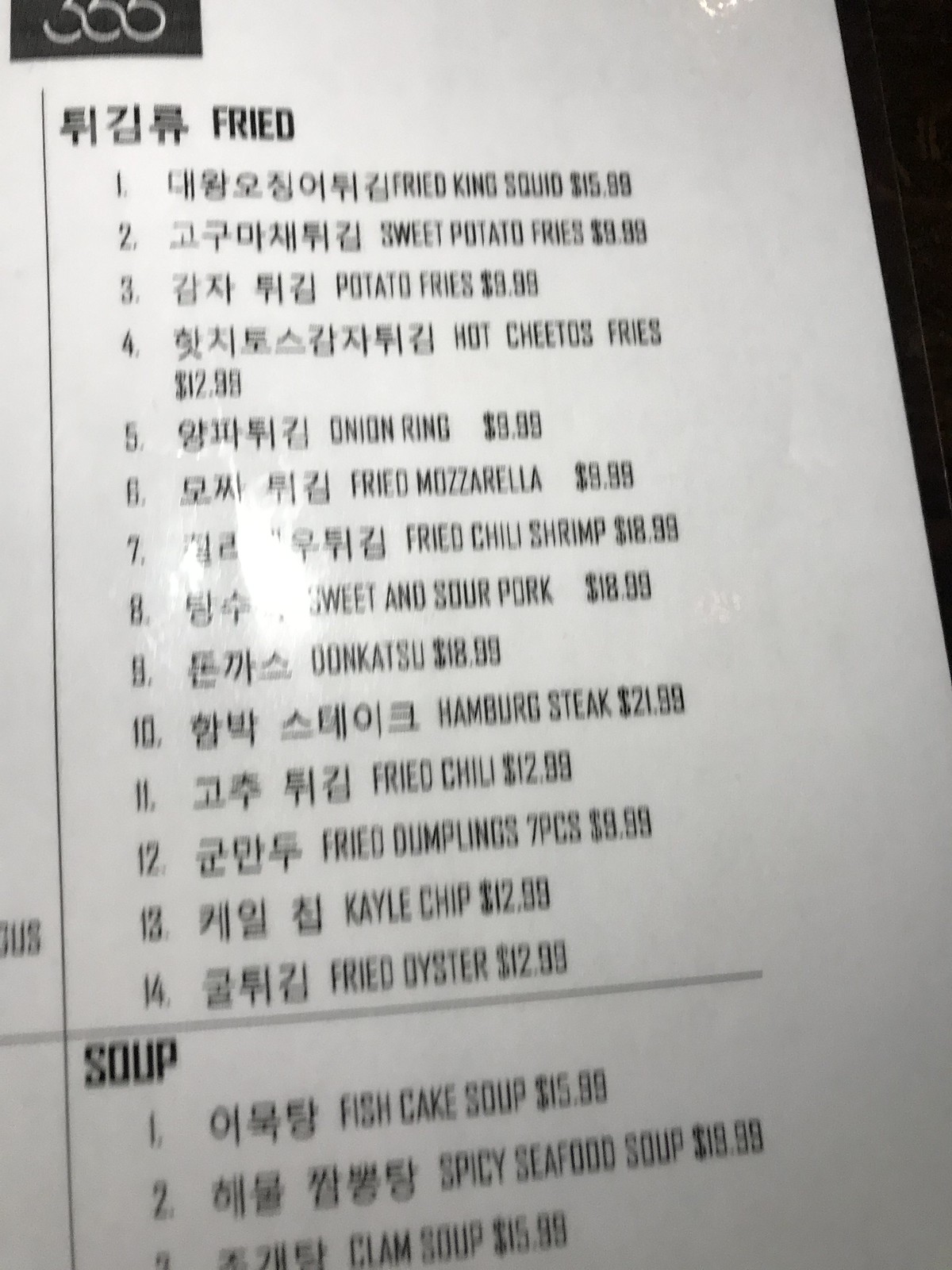This detailed image depicts a black-and-white menu printed on white paper, with the text and logo rendered in black. At the top of the menu, there is an unclear numeral that might read 355, 333, or 555. The menu is bilingual, featuring both an Asian language and English.

Under the section labeled "Fried," the following items are listed:
- Fried King Squid
- Sweet Potato Fries
- Potato Fries
- Hot Cheetos Fries
- Onion Ring
- Fried Mozzarella
- Fried Chili Shrimp
- Sweet and Sour Pork
- Don Katsu
- Hamburg Steak
- Fried Chili
- Fried Dumplings (seven pieces)
- Kale Chip
- Fried Oyster

The prices in the "Fried" section range from $9.99 to $21.00.

Under the "Soup" section, the following varieties are mentioned:
- Fish Cake Soup
- Spicy Seafood Soup
- Clam Soup

The prices for the soups are $15.88, $18.88, and $15.88, respectively. The menu provides a variety of fried and soup options, appealing to those who appreciate diverse culinary choices.